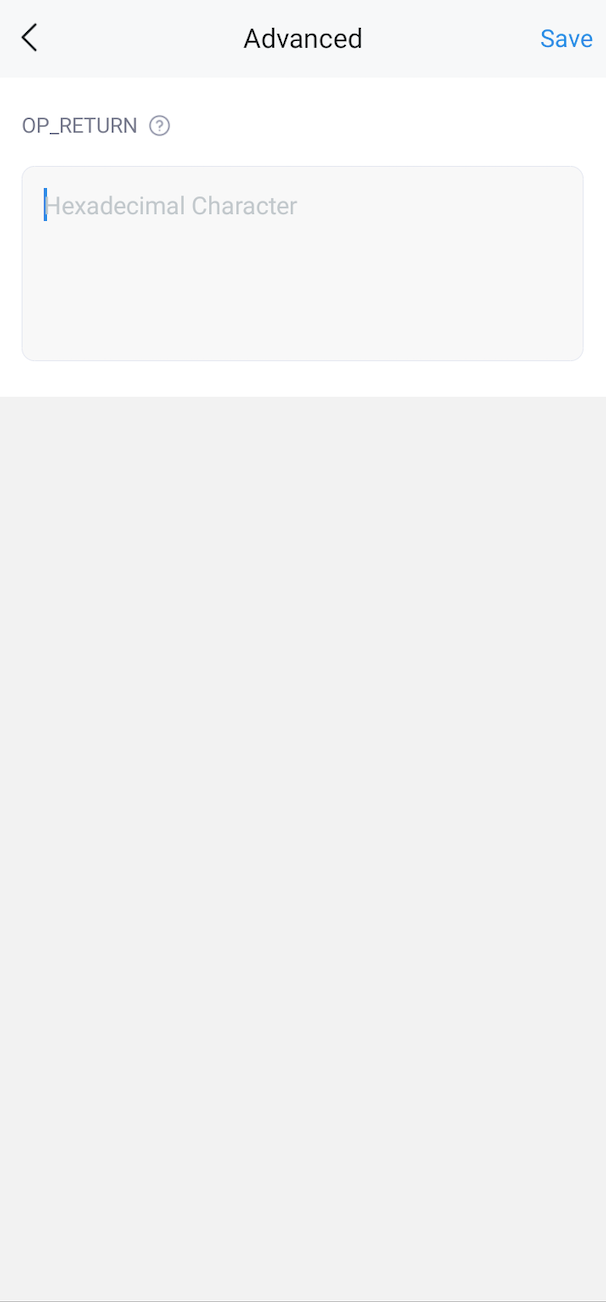This is a detailed caption for the image described:

---

A screenshot taken from a smartphone, possibly an Android or iPhone, features a primarily white background with no visible borders, although parts of the phone are discernible. The screenshot reflects the phone’s full-width display. At the very top, a gray rectangular banner spans the width of the screen. On the left side of the banner, there is a left-pointing arrow icon. Central to the banner, the word "Advance" appears in standard font, without any bolding. On the right side of the banner, the word "Save" is highlighted in blue, suggesting it is a clickable option.

Below the banner, the term “OP_RETURN” appears in all capital letters, followed by an underscore. To the right of this term, there is a faint question mark enclosed within a circle. 

Next, a rectangular box with curved edges is positioned below, which is shaded slightly and contains the text “Hexadecimal character.” This text is also faded, and a prominent blue cursor is positioned at the end of the text within the box.

Further down, there is a small gap leading to a large, grayed-out area with pointed edges, completing the lower section of the screenshot.